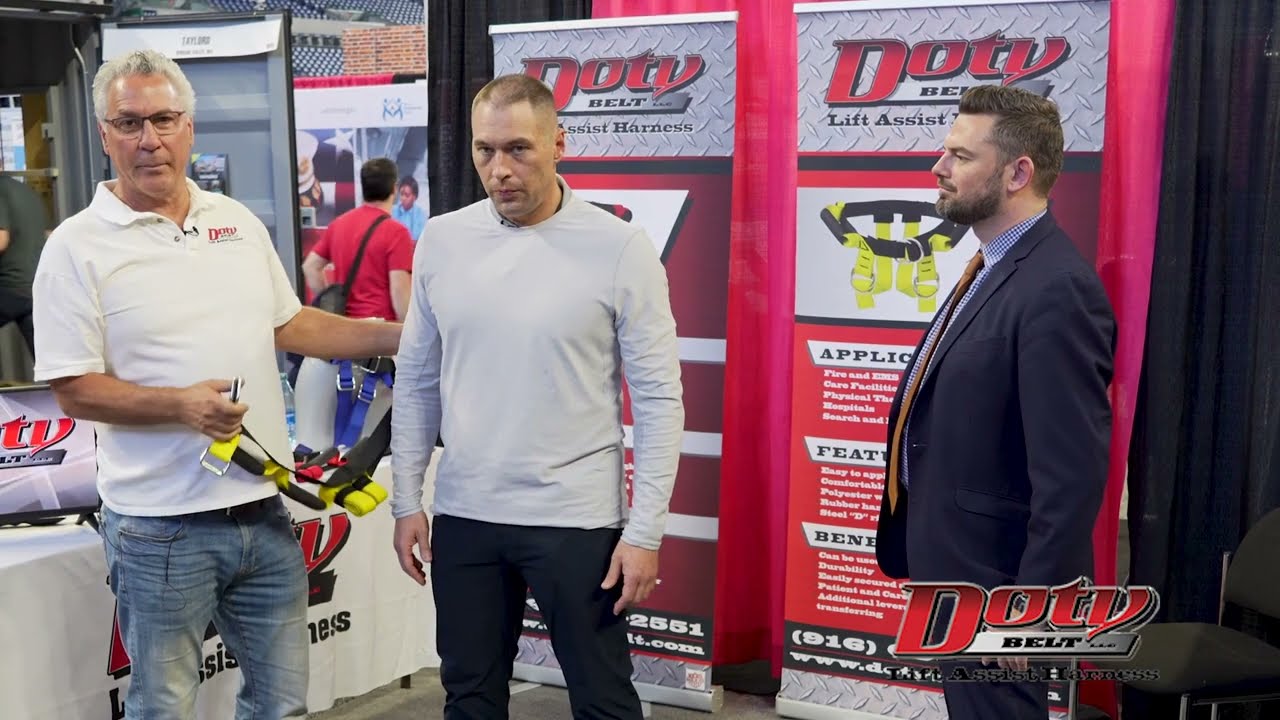In the image, three men are positioned around a booth at a trade show, focused on demonstrating a yellow and black lift assist harness known as the "DOTY Belt." The man on the left is older, with white hair and glasses, dressed in a white polo shirt featuring a company logo and blue jeans. He holds the harness and appears ready to demonstrate it to the man in the middle. This man, wearing a light gray long-sleeved shirt and black pants, stands still with a serious expression. The third man, positioned to the right, is observing the demonstration. He is dressed in a navy blue suit with a mustard tie and a plaid blue and white button-down shirt, sporting a neat beard and styled hair. Behind them are tall vertical signs with the brand and product name "DOTY Belt Lift Assist Harness" in red and black lettering. Additional activity is visible in the background, suggesting a bustling convention or trade show environment. A man wearing a red t-shirt and carrying a bag can be seen among the crowd, adding to the lively atmosphere.